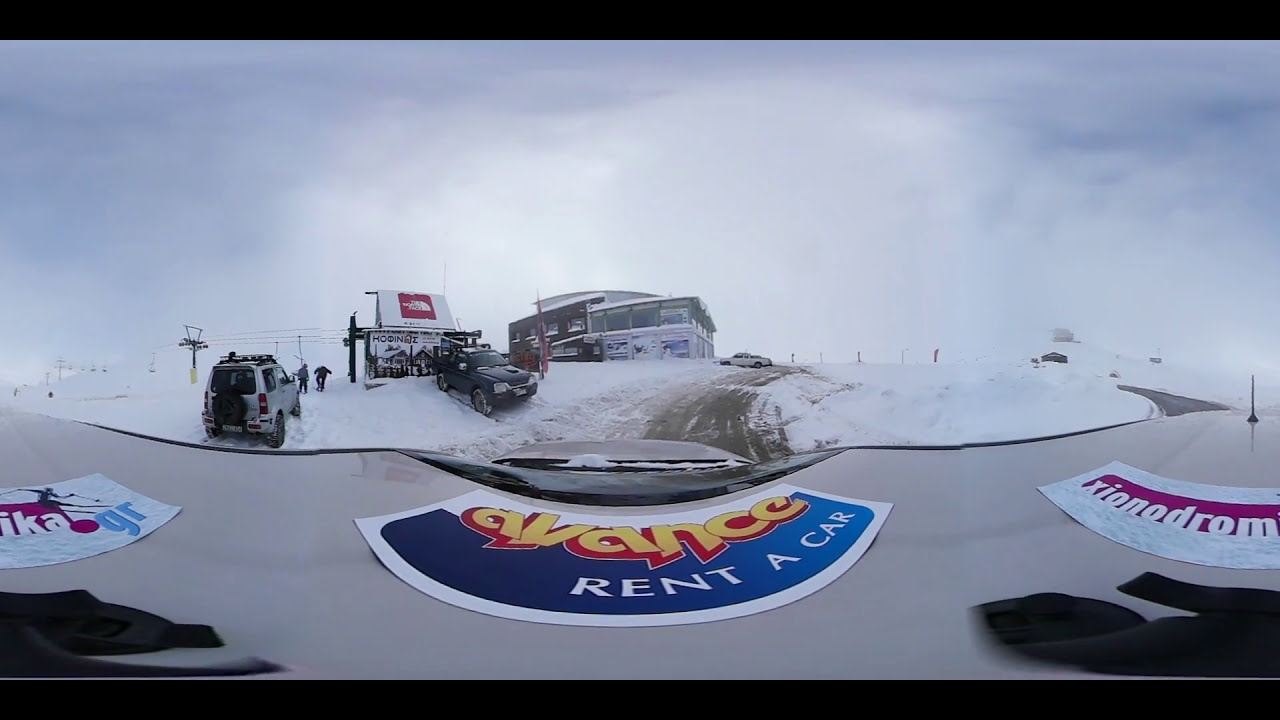This image captures a detailed winter scene, seemingly taken with a fisheye lens mounted on the hood of a white vehicle. The view reveals a snow-covered road ahead, flanked by high snowbanks on both sides. In the foreground, a blue sticker with yellow text reading "Avalanche Rent a Car" and additional white text is visible on the vehicle’s roof.

On the left side of the road, multiple SUVs are parked near a small structure with a triangular roof, adorned with The North Face branding. Behind this, a large building with extensive glass windows and a dark facade spans the scene, resembling a ski lodge. To the right, another building with large windows runs parallel to the road, enhancing the sense of a resort area.

In the distance, a ski lift or gondola system is visible against the cloudy, overcast sky, reinforcing the notion of a high-altitude ski resort. Several warmly dressed individuals navigate the scene, adding to the bustling yet isolated winter atmosphere.